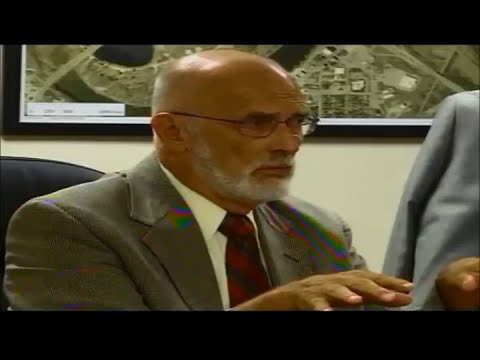The photograph depicts a serious-looking older man in an office setting, possibly engaged in a business meeting. He appears to be in his 70s, characterized by light brown skin, a white beard, a white mustache, and glasses. He is mostly bald with a hint of gray hair at the back. Sitting in a black office chair, he is donning a light brown business suit paired with a white collared shirt and a red and black tie. The man is gesturing with both hands raised in front of him, his mouth closed, almost giving a slight frown. 

To his right, a gray suit jacket hangs on the back of another chair. The background features a crude city map on the wall, showcasing a river and buildings, likely a satellite photograph of some parts of the Earth. The image has a thin black header and footer, possibly indicative of it being taken from an older television screen due to its slight pixelation and discoloration. We see about three-quarters of the man's face as he looks towards the right-hand side of the screen.